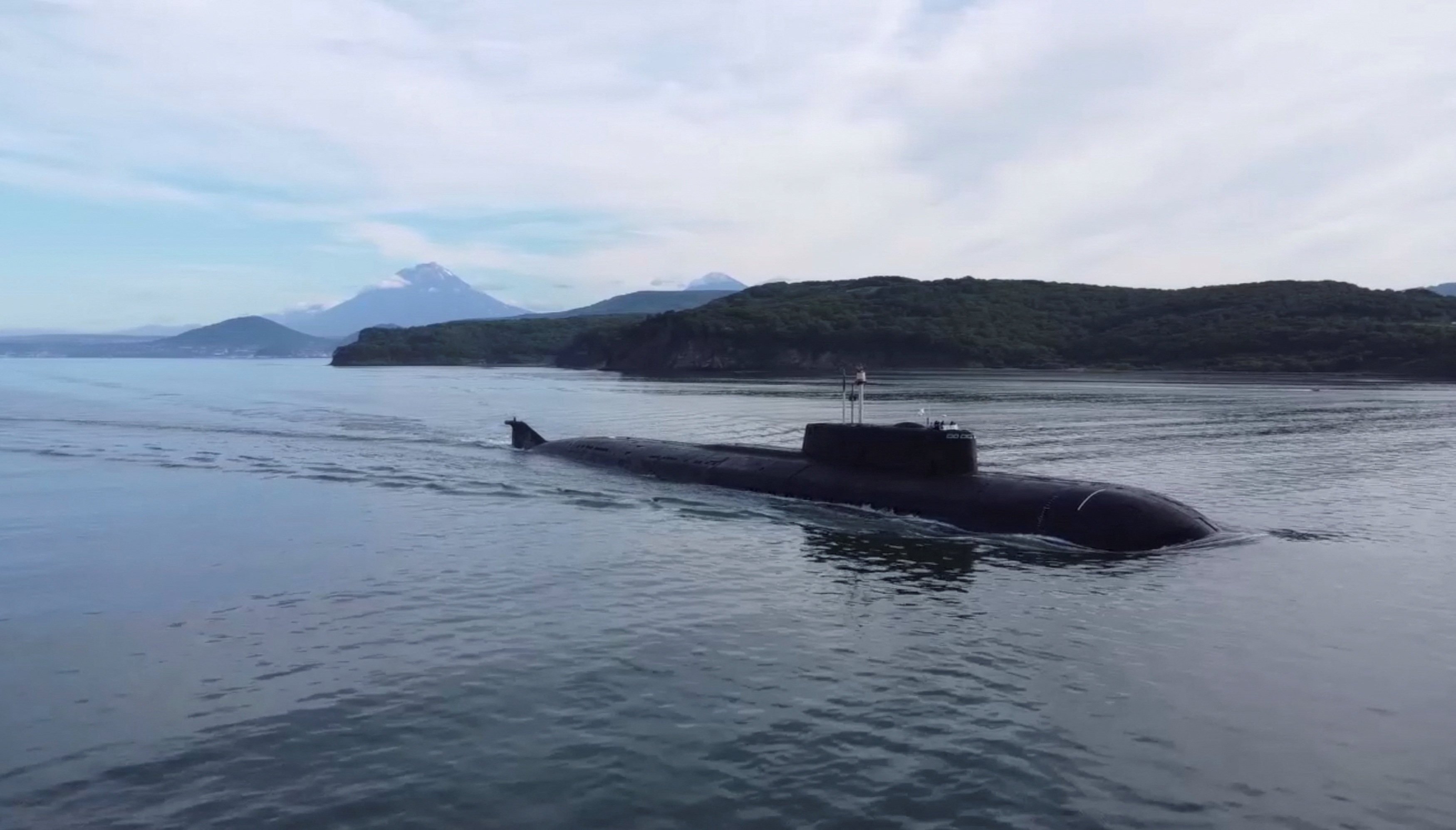In the image, a black submarine is seen partially submerged in what appears to be an ocean or large waterway, moving to the right, as evidenced by the ripples trailing behind it. The submarine resembles a mechanical whale in its sleek, aquatic form and seems poised for deeper submersion. The water surrounding the vessel varies in color, with a dark black hue on the right and a more bluish tint on the left, likely reflecting the partly cloudy sky above. In the background, random green landmasses and higher mountains, possibly resembling volcanoes, rise from the water. These landforms appear hazy on the distant horizon, with clouds nestled around their peaks. On the right side of the image, one of the islands is densely covered with trees, adding to the natural scenery. This daylight shot captures both the mechanical marvel of the submarine and the serene, cloud-dotted landscape surrounding it.